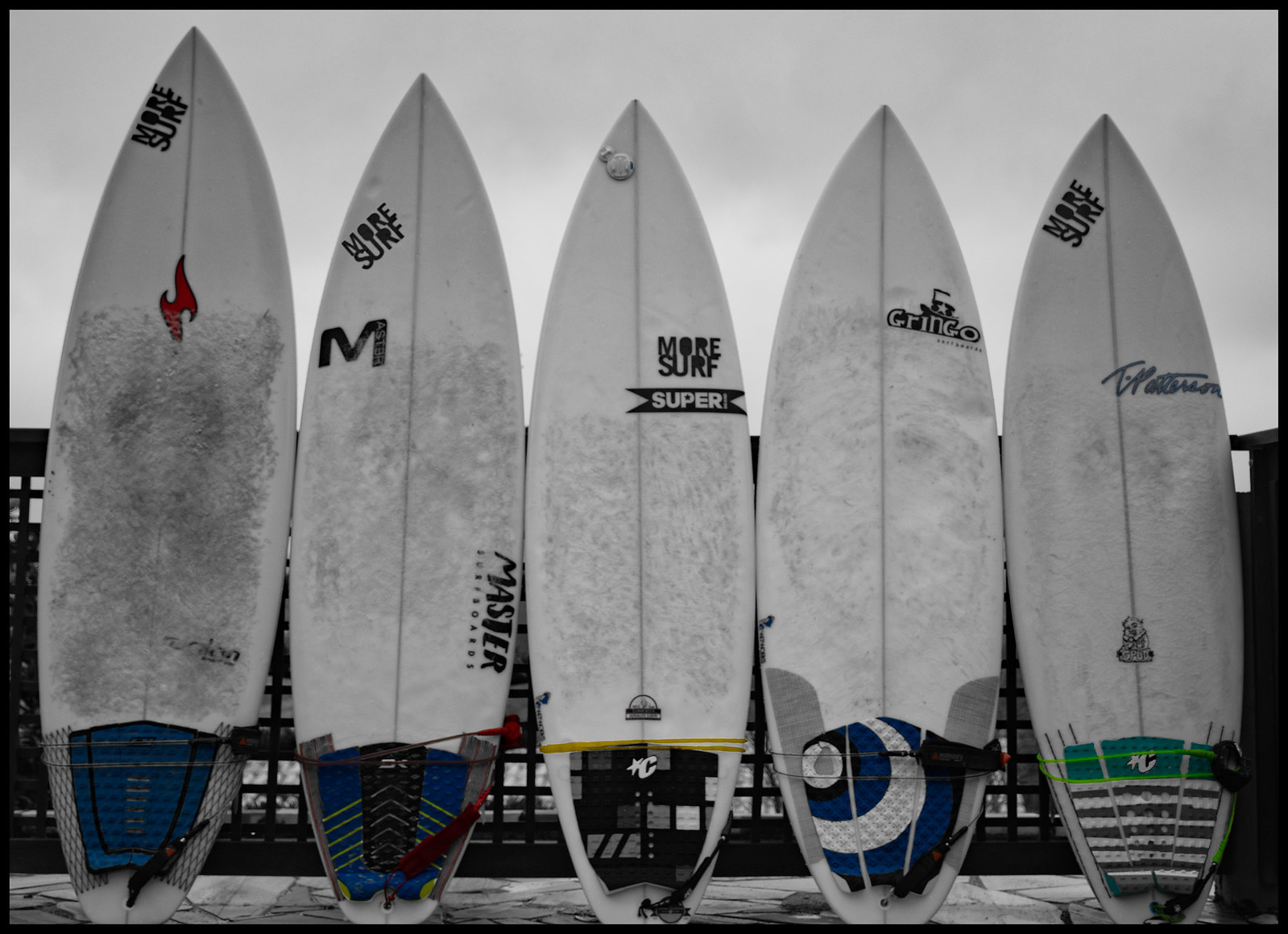This horizontal photograph captures five upright surfboards leaning against a geometric black wrought iron fence on a stonework ground, possibly a boardwalk. Four of the surfboards are branded by the company MorSurf, showcasing the name in the upper left corner of each board. The fifth surfboard, positioned fourth from the left, bears the brand Gringo with a distinctive hat logo. The boards have varying designs at their bases: the two leftmost boards feature blue patterns, the middle board displays a unique black plaid pattern, the fourth board includes a blue and white abstract design, and the rightmost board flaunts green, white, and reddish stripes along with a little animal decal at the bottom. The rightmost MorSurf board is also adorned with a signature. The sky above is grey and cloudy, adding a contrasting backdrop to the vibrant surfboards.